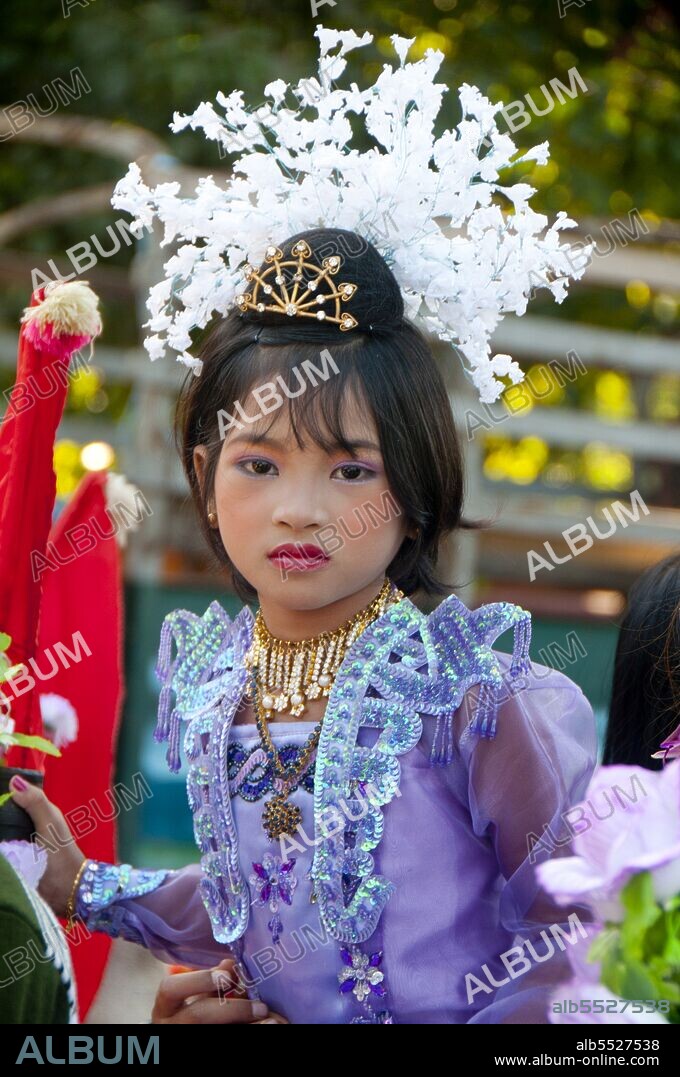In this photograph, a young girl, who appears to be of Asian descent and around seven to ten years old, sits gracefully in a vibrant, ornate costume. Her attire features a light purple dress adorned with sequined ruffles, intricate beading, and sheer long sleeves with embellished cuffs. The dress, highlighted by lace and sparkles, evokes a sense of cultural richness. She wears a heavy gold necklace complemented by another necklace with a gold pendant. Her dark brown hair is crowned with a gold and pearl tiara, from which a bouquet of white flowers artfully fans out. Her piercing gaze is enhanced by fuchsia pink lipstick and purple eye shadow, and her red fingernail polish adds a pop of color. Dangling on the left side of the image are red scarves or possibly flags, adding a splash of color to the blurred background. Additionally, a watermark reading "ALBUM" is faintly visible across the photo.